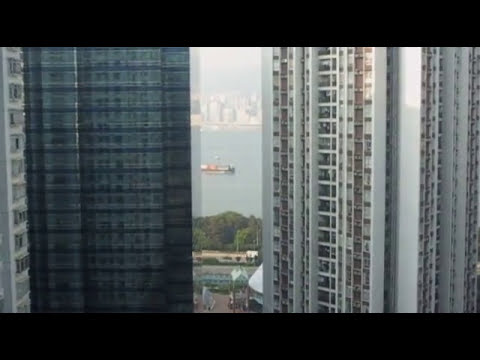This image captures a detailed panoramic view from within one multi-story building, looking across to two distinct neighboring skyscrapers. The building on the left is characterized by its reflective black, glass-dominated facade, giving it a sleek, modern look, while the building on the right stands out with its stark white exterior, dotted with numerous balconies and uniform windows, suggesting a residential use. Nestled between these towering structures, a spacious play area with vibrant playground equipment and verdant trees can be seen at floor level. In the distance, through the gap created by these skyscrapers, a serene bay or river emerges, its gray waters hosting a horizontal cargo ship. Beyond the water's edge, a distant skyline of additional buildings stretches toward the horizon, creating a layered, urban landscape that melds natural and architectural beauty. Black strips border the top and bottom of the image, framing this complex, expansive scene.